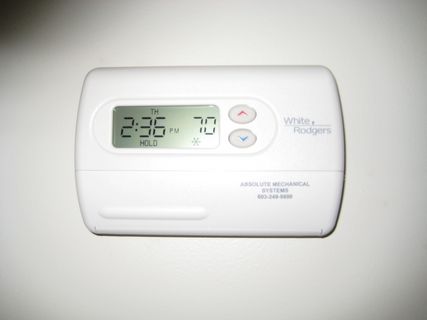The photograph captures a thermostat installed on an unadorned white wall. The thermostat has a rectangular shape with smooth, rounded edges and corners. It prominently features a small LCD screen. On the right side of the device, the manufacturer's name, "White Rodgers," is clearly visible. Below the manufacturer's name, there are additional writings that are not legible.

At the center of the thermostat are two oval buttons: a red one with an upwards arrow, and a blue one with a downwards arrow, presumably used for adjusting the temperature settings. The LCD screen displays essential information, including the current time "2:36 p.m.," the day "Thursday," and the word "Hold." Adjacent to this, the screen shows the number "70," likely indicating the current room temperature or the temperature setting.